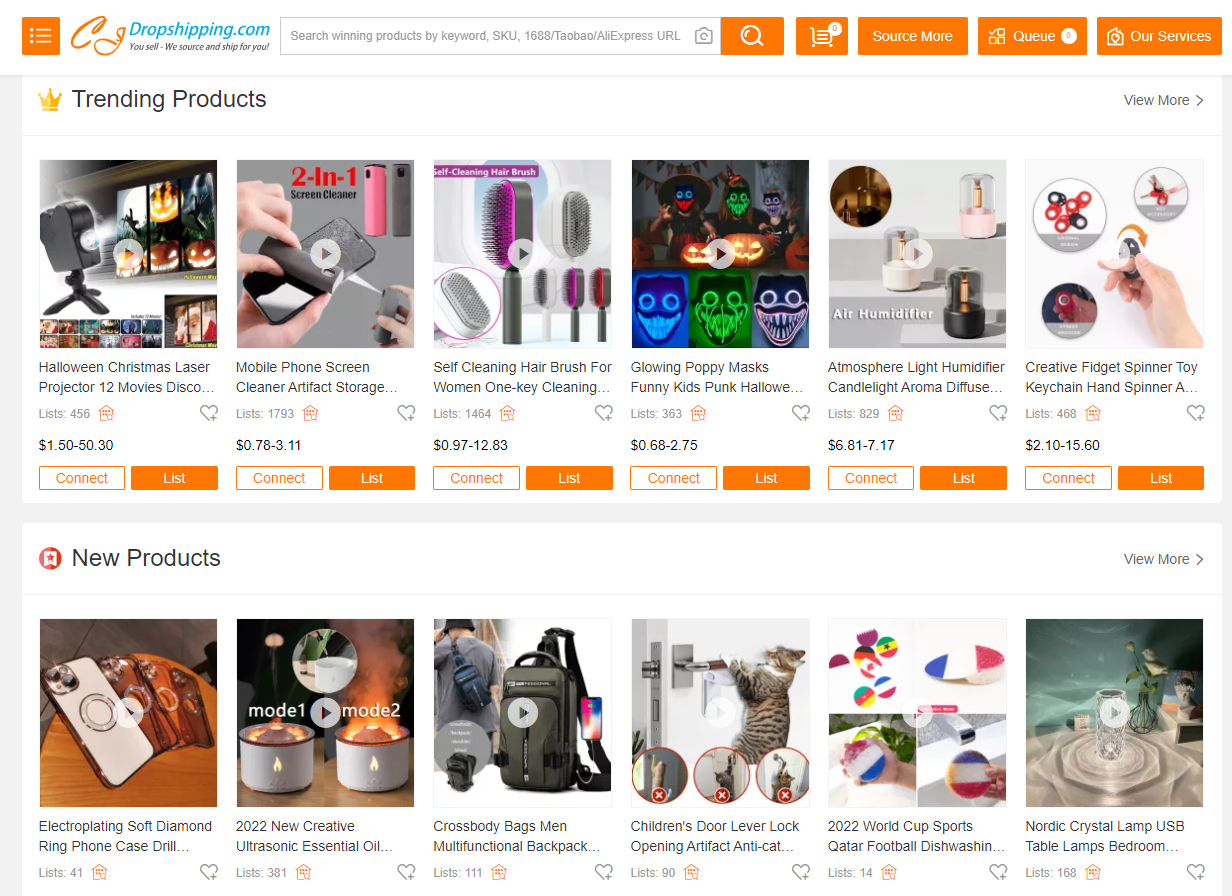The image features the homepage of dropshipping.com, a site that appears similar to Wish, characterized by an orange and white color theme. The page showcases a variety of products with diverse price ranges tailored to different buying needs. At the top, a trending section includes items like a Halloween Christmas laser projector with 12 movies, priced from $1.50 to $50.30 USD. Other trending products include a creative fidget spinner toy, an atmosphere light humidifier, glowing poppy masks, a self-cleaning hairbrush for women, and a mobile phone screen cleaner artifact. Prices for these items vary widely, with some, like the hairbrush, ranging from $0.97 to $12.00 USD, while others maintain an average of $3.00 to $4.00 USD.

Additionally, the site features a category for new arrivals, with items such as a trending soft diamond ring phone case drill, a 2022 new creative ultrasonic essential oil diffuser, a crossbody book bag, a treasured door lever lock, a 2022 World Cup-themed sports photograph football dishwashing sponge, and a crystal nap USB. The platform organizes products into multiple lists, providing customers with an array of options depending on their shopping preferences.